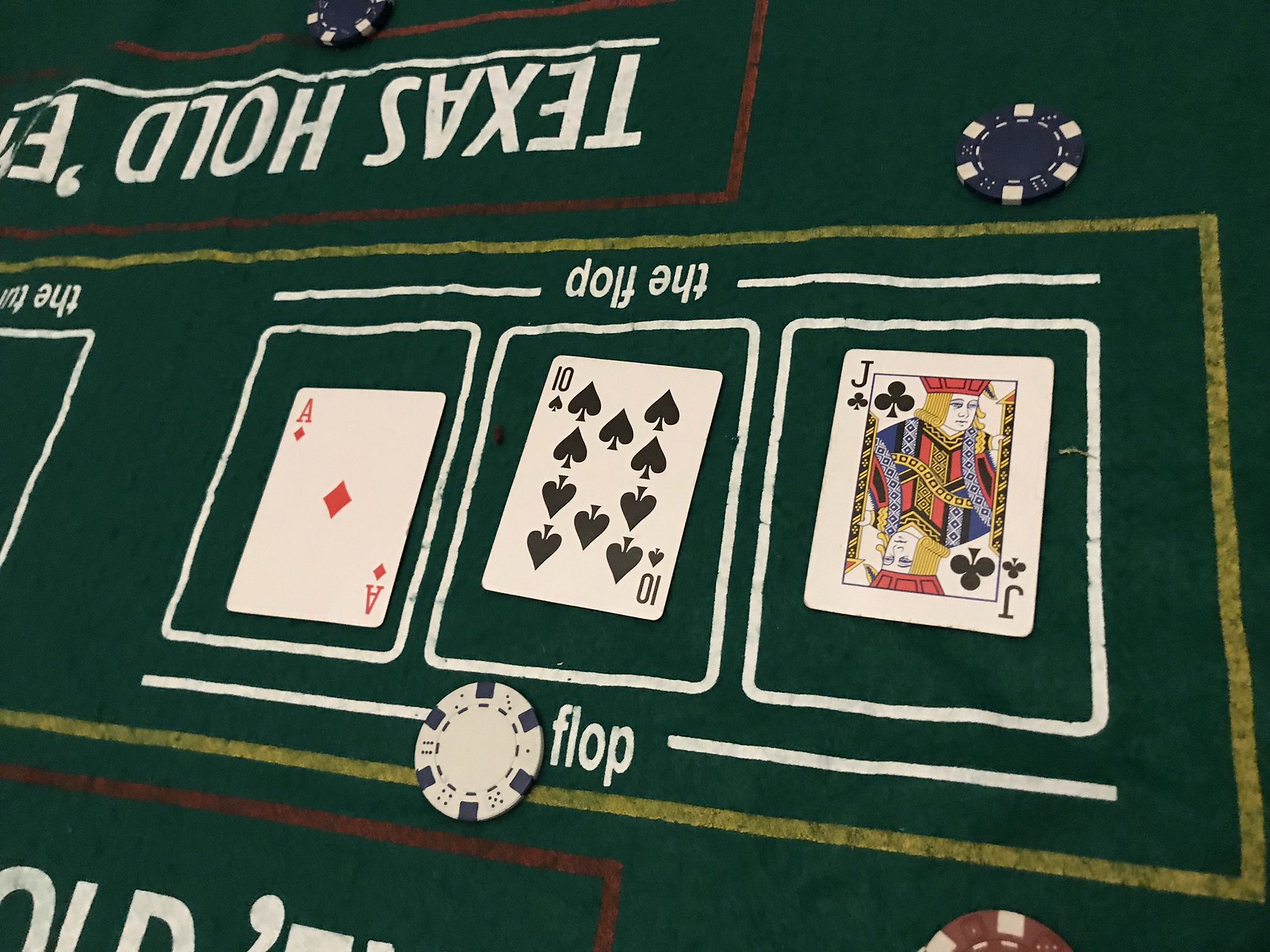In this photograph, a person is engaged in a card game, potentially Solitaire, on a green felt surface. The scene features three prominent cards laid out in the middle: the Ace of Diamonds, the Ten of Hearts, and the Jack of Spades, along with a Joker. Below these cards, a poker chip is visible, displaying the text "Texas Hold'em," although the full phrase is partially obscured. The green felt table, associated with the game, has various poker chips scattered across it, adding to the ambiance of a casual, yet engaging card game session.